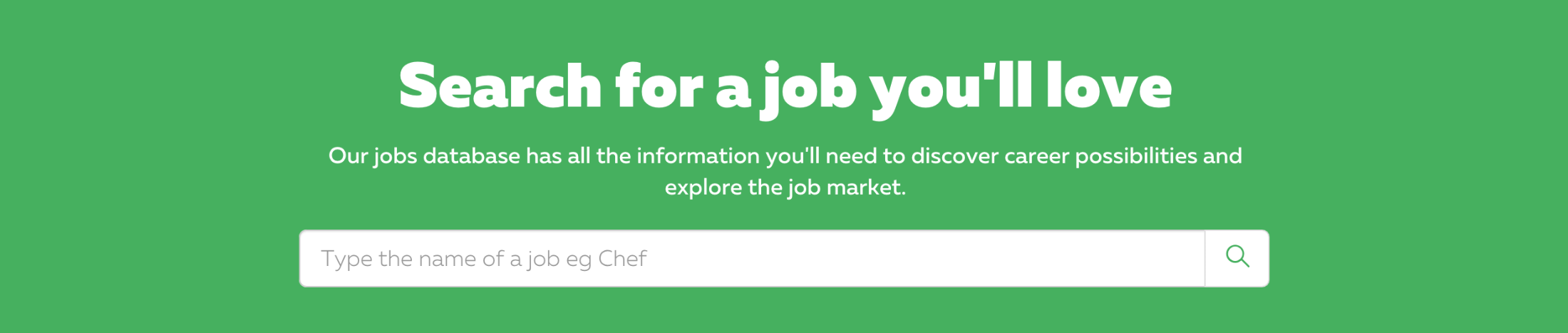In this image, we observe what appears to be a digital screenshot predominantly filled with a solid white background. Centrally positioned in the composition is a prominent, horizontally extended green rectangle. This green box encompasses several key elements: At the top, there is bold, block white text which reads, "Search for a job you'll love." Directly underneath, in a smaller font but still centered, the white text states, "Our jobs database has all the information you'll need to discover career possibilities and explore the job market." Below this narrative, still within the confines of the green rectangle, lies a white search bar. Inside the search bar, in light gray text, are the words, "type the name of a job e.g. chef," which serve as a placeholder prompt for users looking to begin their job search.